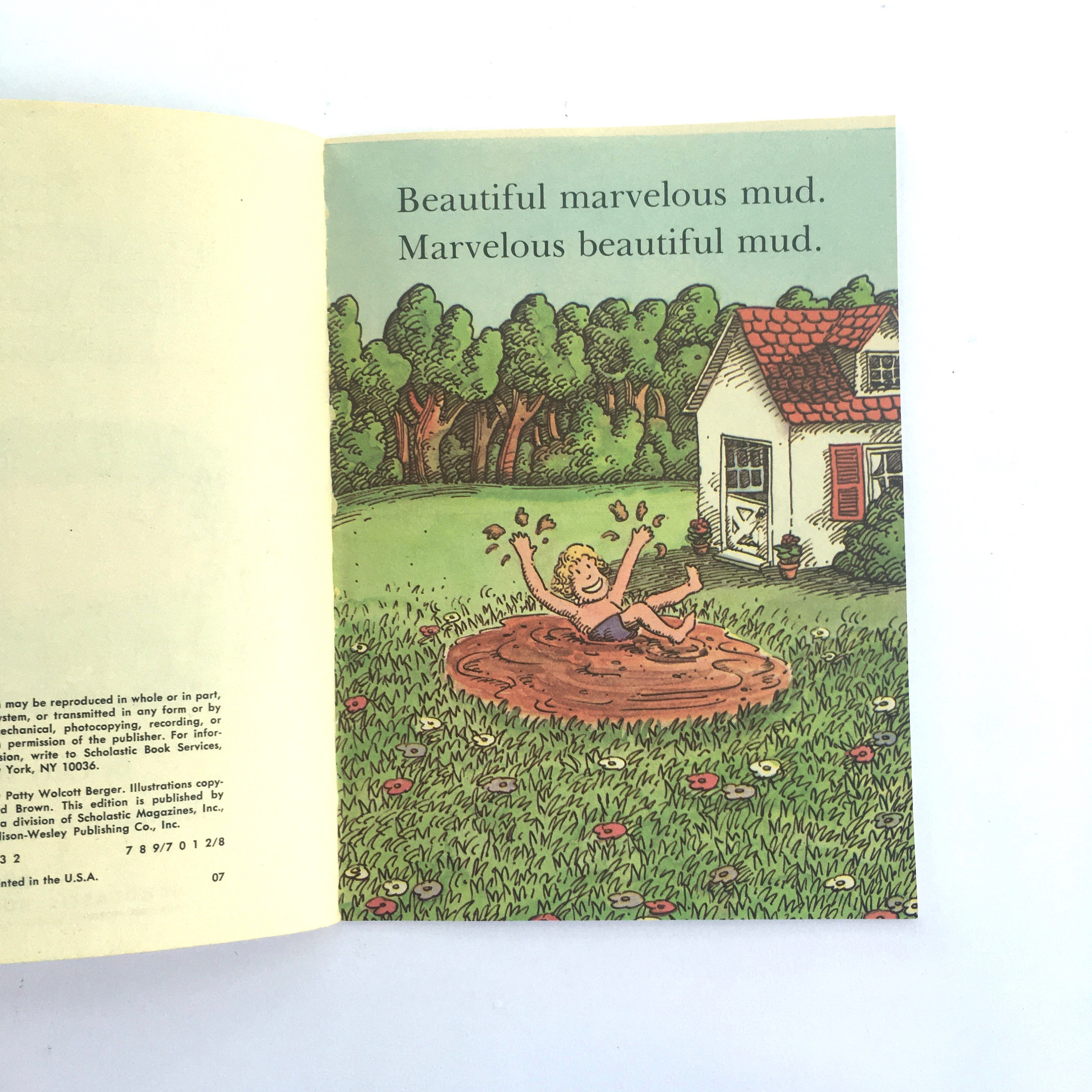The image depicts an open children's book, set against a background that transitions from light blue at the bottom corners to white at the top, partially obscuring the upper right corner. On the left page, which is light yellow and partially out of view, there are two paragraphs of black text at the bottom detailing publishing information, such as "Wesley Publishing Company, Inc.," "Printed in the USA," and a sequence of numbers, "7897012807."

On the right page, there's a vibrant cartoon illustration. The top two lines of black text read, "Beautiful Marvelous Mud, Marvelous Beautiful Mud." Below this, the scene features a young, shirtless boy of Caucasian descent with blonde hair and wearing dark blue or black shorts. He is joyfully jumping into a mud pit, splashing mud into the air. Surrounding the mud pit is green grass dotted with red, white, and light black flowers. To the right of the boy stands a simple white house with a red tile roof and a shed door, accompanied by a small bush. In the background, there's a line of trees that completes the picturesque, playful setting.